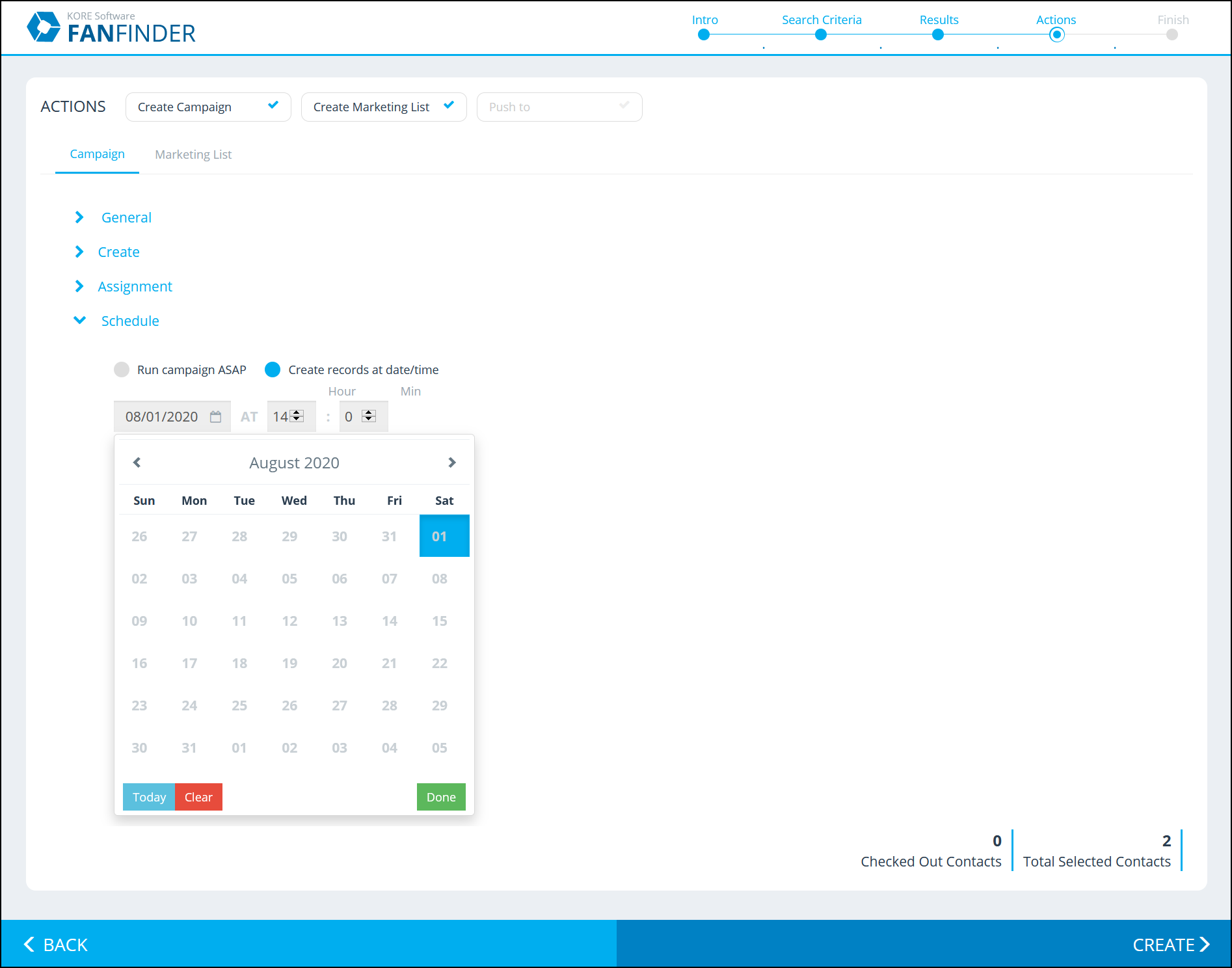In the image, we're viewing a screen interface labeled "Fan Finder" in blue text at the top left corner. To the right, there are five navigational words: "Intro," "Search Criteria," "Results," "Actions," and "Finish." The first four words are highlighted in blue with corresponding blue dots, indicating progress, while the word "Finish" is in gray with a gray dot, showing it is not yet completed.

Below this section, the label "Actions" is visible along with two options: "Create Campaign," which is highlighted in light blue, and "Create Marketing List," in gray. Further down, there are four light blue options: "General," "Create," "Assignment," and "Schedule."

Centered below these options, there's a calendar set to August 2020, which can be adjusted by date, hour, and minute. The calendar dates start on Sunday the 26th and end on the 5th of the following month, or possibly two months ahead. Days of the week from Sunday to Saturday are abbreviated and displayed in black text. The top right cell of the calendar is a blue square marked "01."

Additionally, there are three function buttons beneath the calendar: "Today" in light blue, "Clear" in red, and "Done" in green. At the very bottom of the screen, the left side shows a turquoise "Back" button, while the right side features a blue "Create" button.